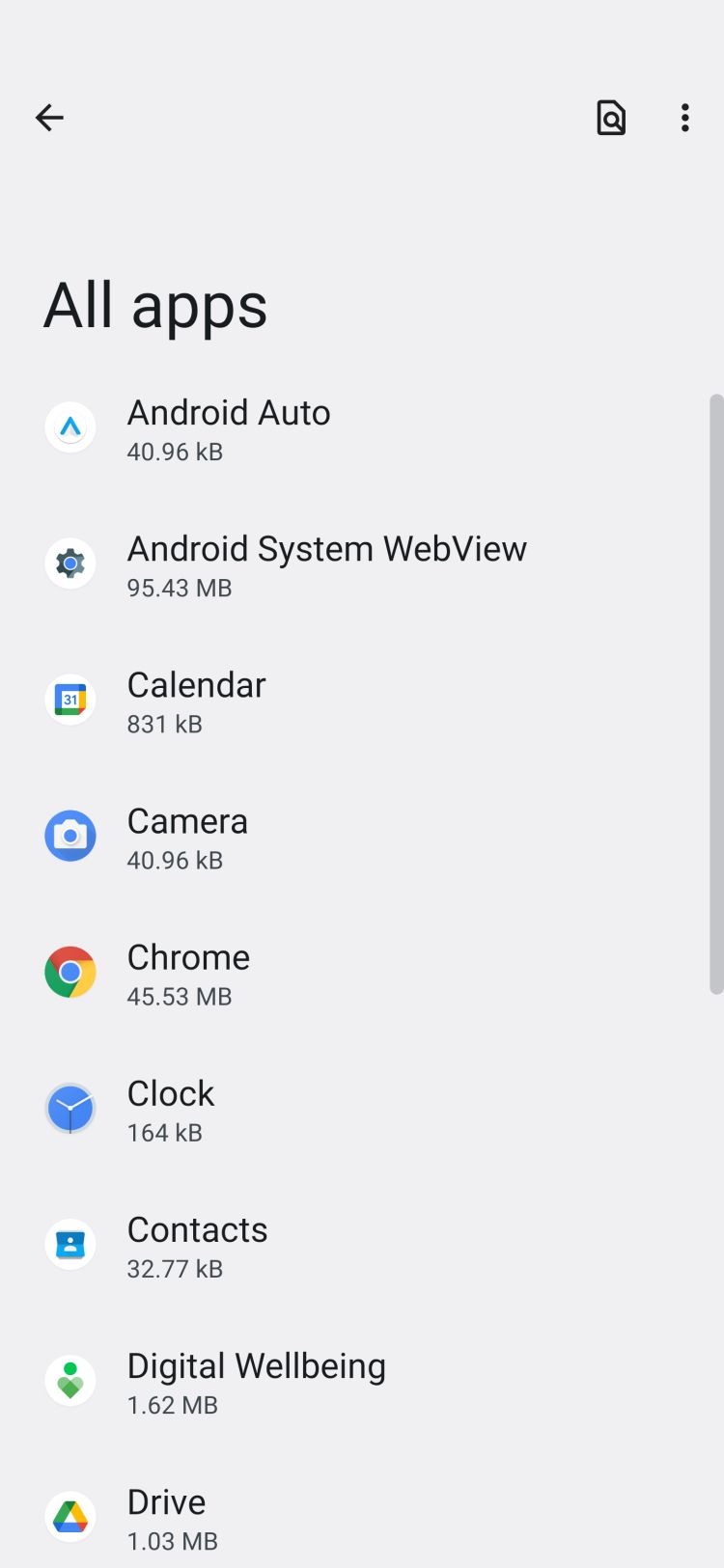The image displays a screenshot of a website interface on a mobile device, evident by the presence of smartphone navigation icons such as a camera icon and three vertical dots on the top-right corner, as well as a back arrow on the top-left. Below these icons is the title "All apps" in bold black font, indicating that the current screen shows a list of applications.

The visible app list begins with:

- Android Auto
- Android System WebView
- Calendar
- Camera
- Chrome
- Clock
- Contacts
- Digital Wellbeing
- Drive

These applications are organized in alphabetical order with their respective icons positioned to the left of their names. The interface is predominantly medium gray in color, providing a neutral backdrop allowing the app icons to stand out. 

Notably, the Chrome app icon, with its red, green, blue, and gold colors, and the Google Drive icon with its familiar color scheme, are easily identifiable amongst the gray tones.

On the right side of the screen, there is a vertical scrolling bar colored in gray, which implies that the user can scroll up or down to view additional apps beyond the visible list.